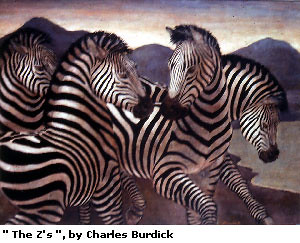The image is a drawing or computer-generated picture titled "The Zs" by Charles Burdick. It depicts four zebras with black and white stripes, positioned closely together. The two zebras in the center have their heads almost touching, inches apart, and appear to be facing each other with legs raised as if in motion. The other two zebras are positioned on either side, with their heads tilted downward. The background shows blue-colored mountains with a partially visible sky that exhibits shades of yellow, light brown, beige, and a touch of blue. The picture is rectangular, roughly 2 by 2 inches in size, and the full bodies of the zebras are not visible, as they are cut off by the picture's corners.